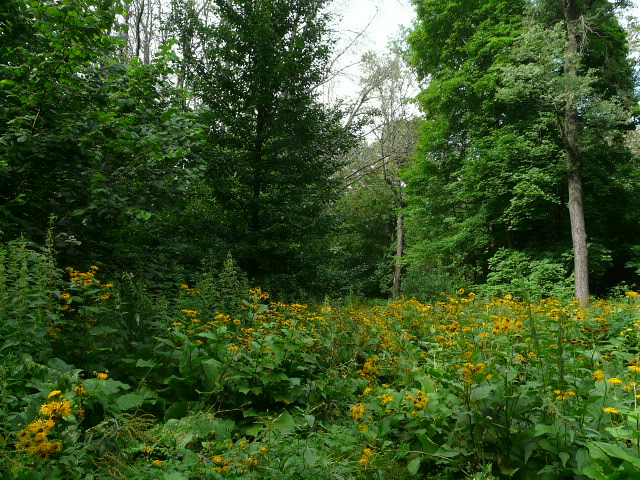This vibrant outdoor photograph captures a lush natural scene bathed in daylight. In the foreground, low-lying plants adorned with dozens of small, yellow flowers—possibly goldenrod—create a dense, almost untouched thicket amidst some reeds. These flowers stand out against the verdant backdrop and give the appearance of an unremarked, pristine area. Behind this floral carpet, an array of very tall, lush green trees forms the background, typical of a thriving forest in summertime. Notably, a single dead tree punctuates the center, its bare branches starkly contrasting against the rich green foliage around it. The sky, visible just above the trees, is a clear bluish-white, adding to the serene, untouched essence of this forested landscape.